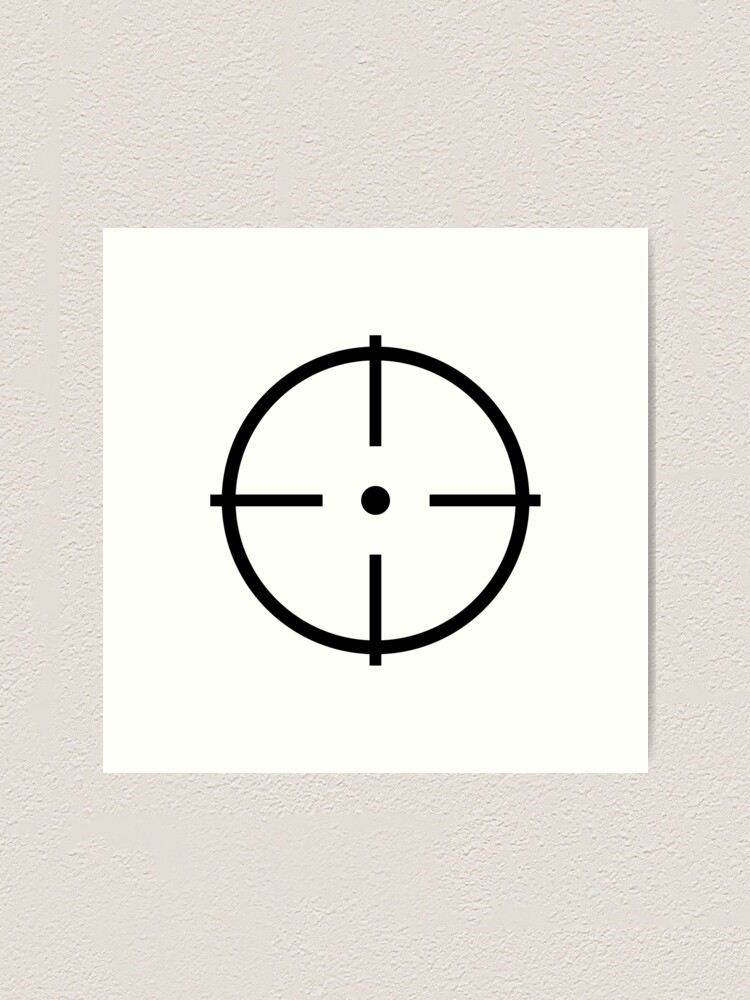The image features a simple yet striking bullseye or target symbol, positioned on a textured white wall that could either mimic stone or be actual stone. Central to the scene is a square piece of white paper mounted on the wall, bearing a meticulously drawn black circle. This circle is adorned with four thick black lines radiating from the cardinal directions—north, south, east, and west—each pointing toward the circle's center. Inside this central circle lies a bold black dot, acting as the bullseye of the design. The composition is clean and straightforward, devoid of any text or additional markings, leaving the focus entirely on the stark, minimalist design of the target symbol.